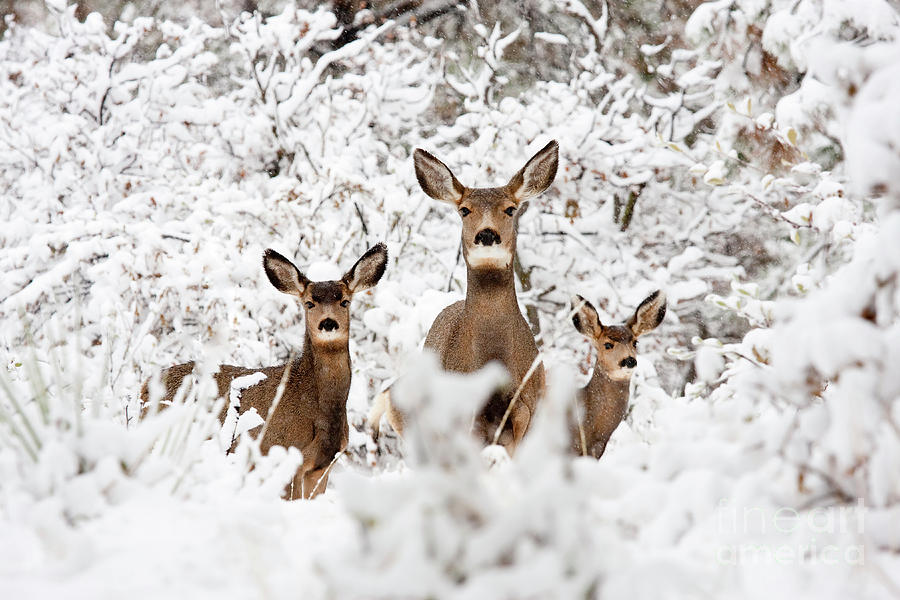In this serene outdoor winter scene, three deer stand together in a snow-blanketed forest. The landscape is draped in a heavy covering of fresh snow, estimated to be two to three inches deep, enveloping the leafless foliage and thicket. The trio is composed of a larger doe and her two smaller offspring, likely twins, all devoid of antlers and clad in brown fur. The doe stands in the center, gazing directly into the camera with her ears perked up, while one fawn mirrors her gaze and the other glances slightly to the side. The snowy setting and the deer's attentive postures create an enchanting, almost magical atmosphere. In the bottom right corner of the image, a subtle, see-through watermark reads "Fine Art America," adding a professional touch without distracting from the natural beauty of the scene.